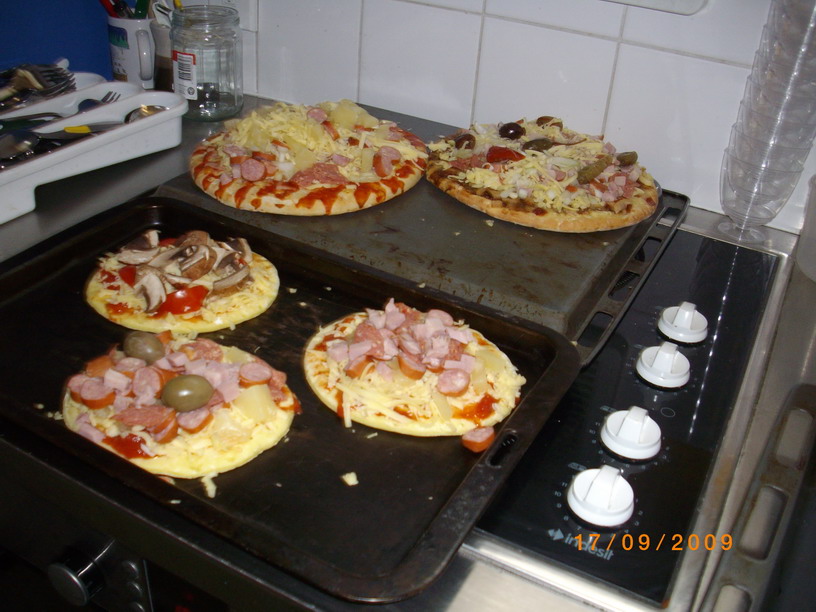This detailed photograph captures a scene in a home kitchen looking down at a black, flat electric stovetop situated beneath a white-tiled wall. At the center of the stovetop lie two black baking sheets positioned horizontally. The first tray, which is upside down, holds two larger pizzas that appear freshly cooked. These pizzas are heavily adorned with pink sausage bits, yellow cheese, black olives, and both green and red peppers.

In front of this, resting on a correctly oriented tray, are three smaller, uncooked pizzas. These pizzas share a base of cheese and red sauce but feature diverse toppings: the one on the left is garnished with onions, red pepper slices, and more cheese; the middle pizza boasts olives, sausage bits, and additional cheese; while the frontmost pizza, clearly showing sausage bits, black olives, and a hint of cheese.

To the left of the stovetop is a white plastic silverware tray brimming with silverware, accompanied by a clear plastic bottle and a white mug which seems to house various markers and screwdrivers. Further features include a date stamp "17-09-2009" in orange numerals in the lower right corner, and a cluster of what seem to be transparent plastic ice cream cups stacked at the back of the stove. The overall composition paints a vivid and bustling image of a kitchen in active use.